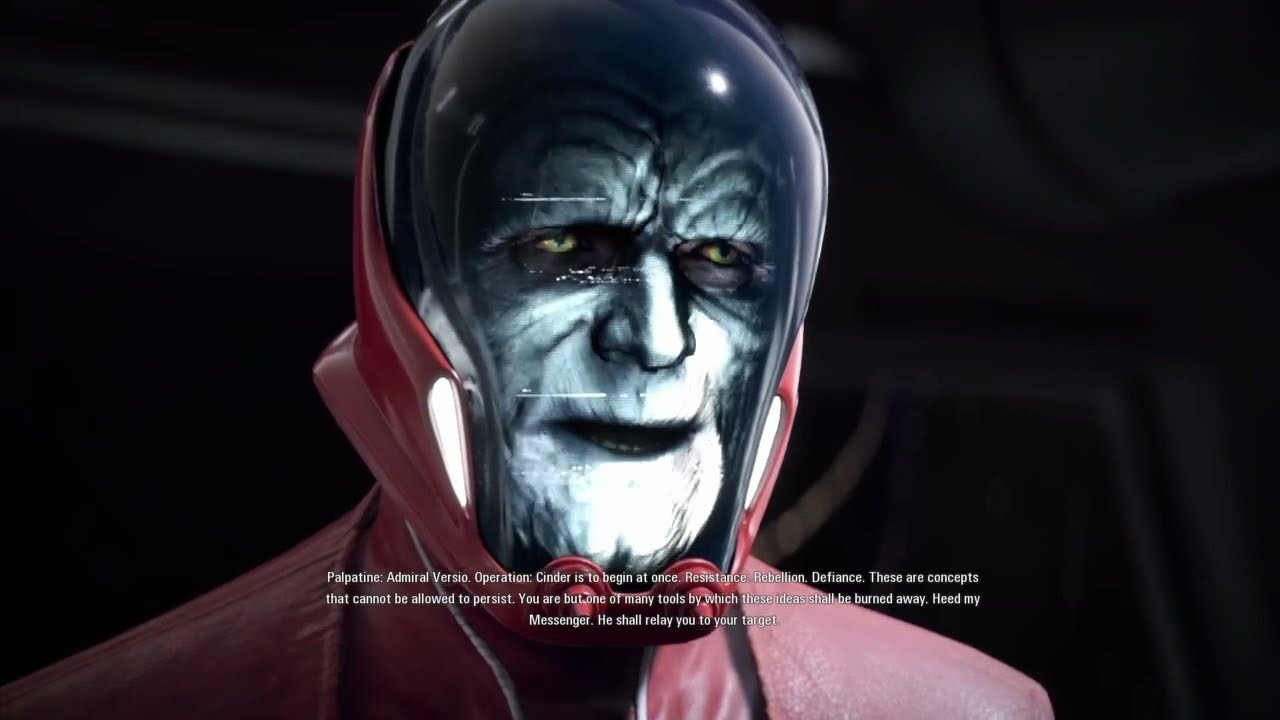In the image, a cartoon character clad in a red suit is visible from the shoulders up. His head is encased in a helmet, with the top portion red and the face cover made of transparent glass. Behind the glass, his face, which is aged with many wrinkles, has a ghostly and blue-gray appearance, almost resembling an alien. Notably, the character has strikingly green eyes. The background is a very dark, almost black, setting. At the bottom of the image, small white text reads: "Palpatine: Admiral Versio, Operation: Cinder is to begin at once. Resistance, Rebellion, Defiance—these are concepts that cannot be allowed to persist. You are but one of many tools by which these ideas shall be burned away. Heed my messenger; he shall relay you to your target." This scene appears to be a still from a Star Wars video game, featuring Emperor Palpatine delivering a commanding message.